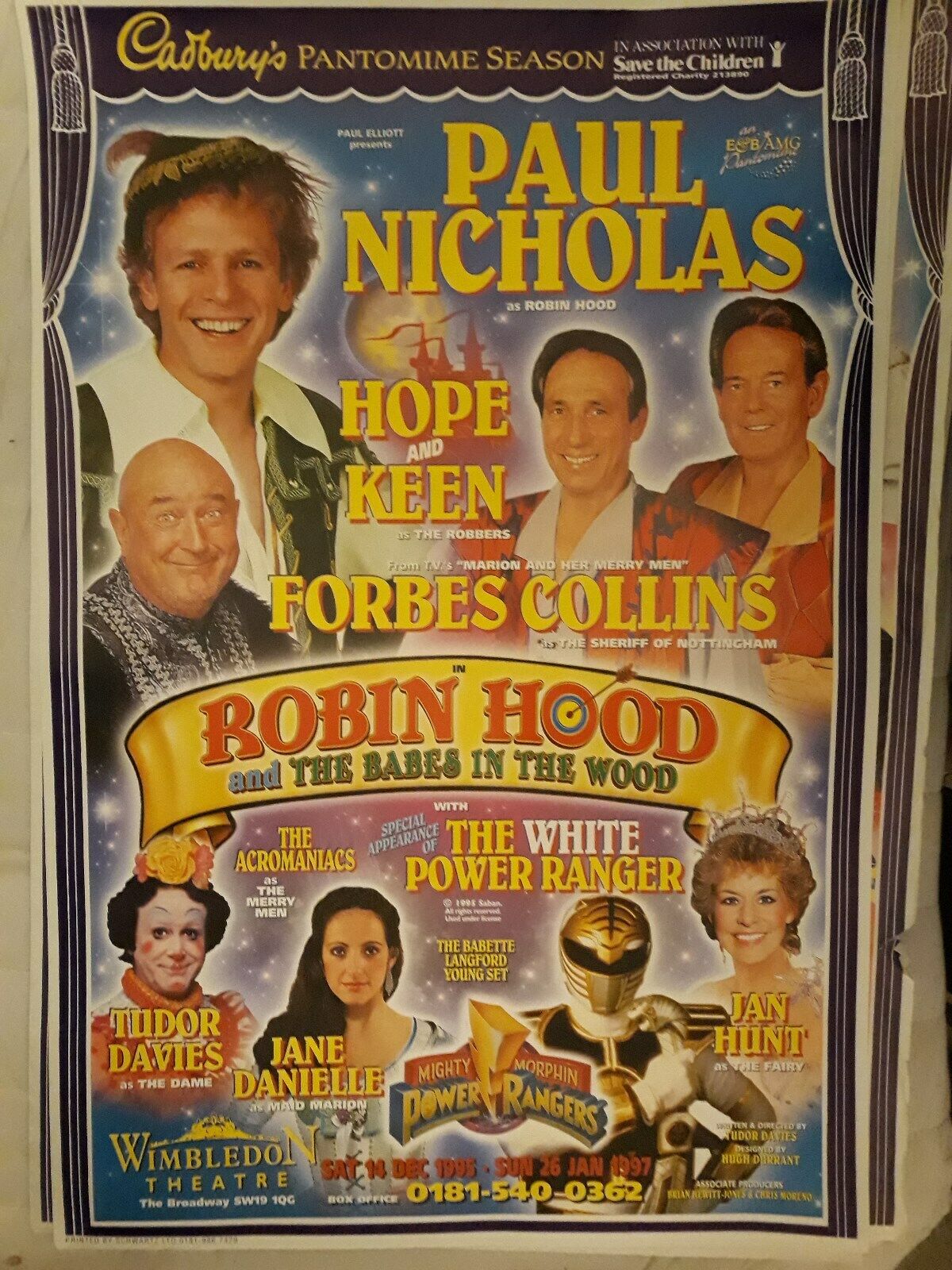This vibrant poster from the 70s or 80s, showcasing Cadbury's pantomime season in association with Save the Children, invites theatergoers to the Wimbledon Theatre. The design is framed by a drawn purple curtain, enhancing the lively imagery and festive atmosphere. At the top in bold yellow text, it reads: "Cadbury's pantomime season in association with Save the Children."

The central focus of the poster is the title of the pantomime, "Robin Hood and the Babes in the Wood," with "Robin Hood" prominently displayed in red letters against a yellow banner, where the first "O" is depicted as a target with an arrow. Surrounding this title, the names and faces of the cast are highlighted. Paul Nicholas stars as Robin Hood, pictured in a fitting costume at the top left. Hope and Keen, playing the robbers, smile from next to him, donned in their distinctive outfits. Forbes Collins is depicted as the jolly Sheriff of Nottingham.

Below these, additional cast members are featured, including Tudor Davies as a clown with a flower headpiece, Jane Danielle with flowing brown hair, and Jan Hunt as a fairy, adorned with a crown and royal attire. A special appearance by the White Power Ranger is also noted, adding a modern twist to the traditional pantomime.

At the very bottom of the poster, in bold text, it announces the venue, Wimbledon Theatre, along with additional contact details. The eclectic mix of performers and vibrant visual elements encapsulate the theatrical and enchanting spirit of this pantomime season.